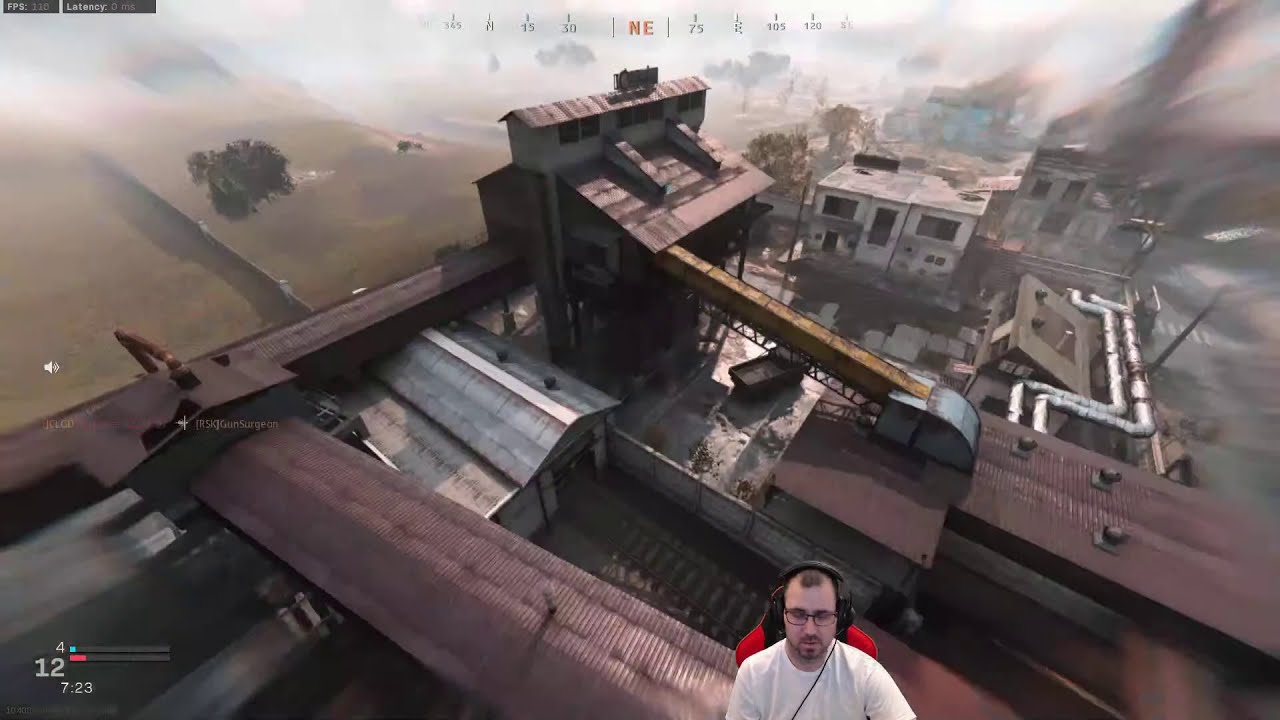This image is a detailed screenshot from a video game, presented in a wide rectangular format. The aerial view reveals an expansive, abandoned industrial complex composed of various outdoor metal structures and intersecting purple metal walkways. On the left side, these walkways intersect near a large green lawn area that blends into a blurry blue sky at the top of the image. The right side mirrors the left with similar structures and a cluster of smaller white buildings in the background, also becoming blurry as they recede.

Centrally placed, slightly to the right and at the bottom of the image, is a man seemingly integrated into the game scene or photoshopped onto it. He is wearing a white t-shirt, glasses, and wired headphones. His brown hair and mustache are visible, and he is seated in a red and black gaming chair. Additionally, a compass indicating "NE" in red letters is located at the top center of the image, with various notches and numbers partially visible. The combination of these detailed elements illustrates a vivid scene where the individual appears to be immersed in or streaming the game, surrounded by a decayed industrial setting that hints at past activity and presence.